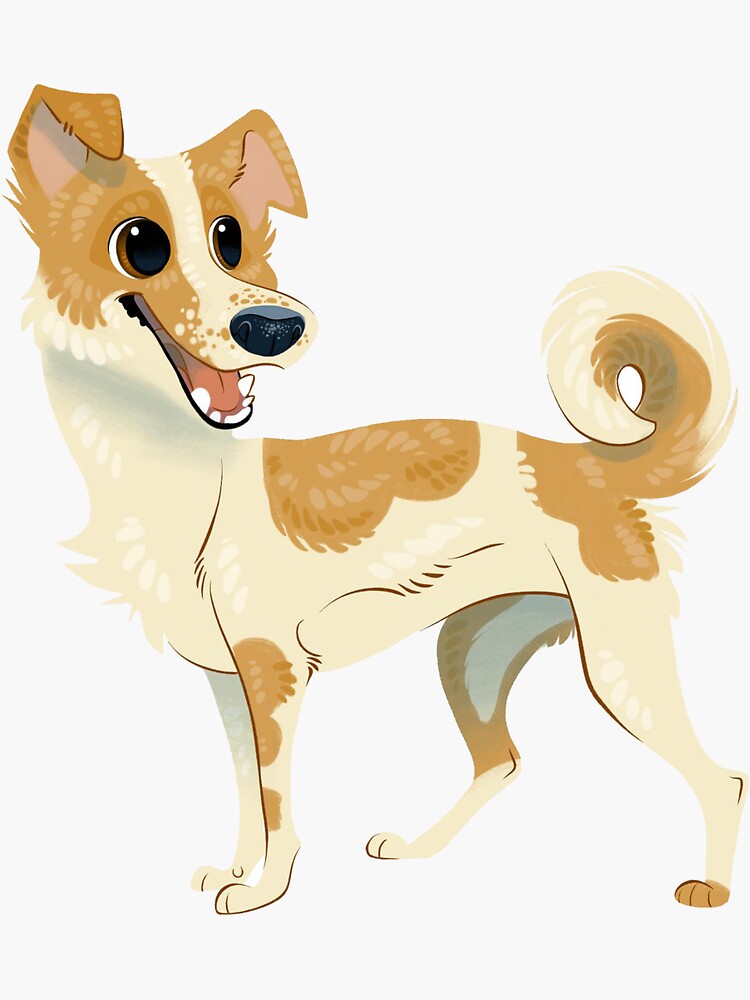This is an illustration of a cartoon-like Canaan dog with an expressive and joyful demeanor. The dog, predominantly cream-colored with an array of brown patches, is shown standing upright on all four legs, oriented to the left but with its head turned back to the right. The attention-grabbing large eyes, adorned with black pupils and brown irises, are directed to the right along with its smiling, open mouth, suggesting a happy expression. The dog has a few white patches, notably on its inner leg visible beneath its body. Its brown markings include spots on its front leg, back leg, and foot, as well as on its tail and back. Distinctly, the dog features a unique facial pattern with brown patches over its ears and face, leaving a cream-colored line from its nose to the head. The ears are floppy, and the tail is lifted and curled towards its head. The background is simple, being white, which emphasizes the dog's detailed and vibrant coloration. There are no additional elements or text in the drawing; it's just the contented dog seemingly looking back at something with curiosity.